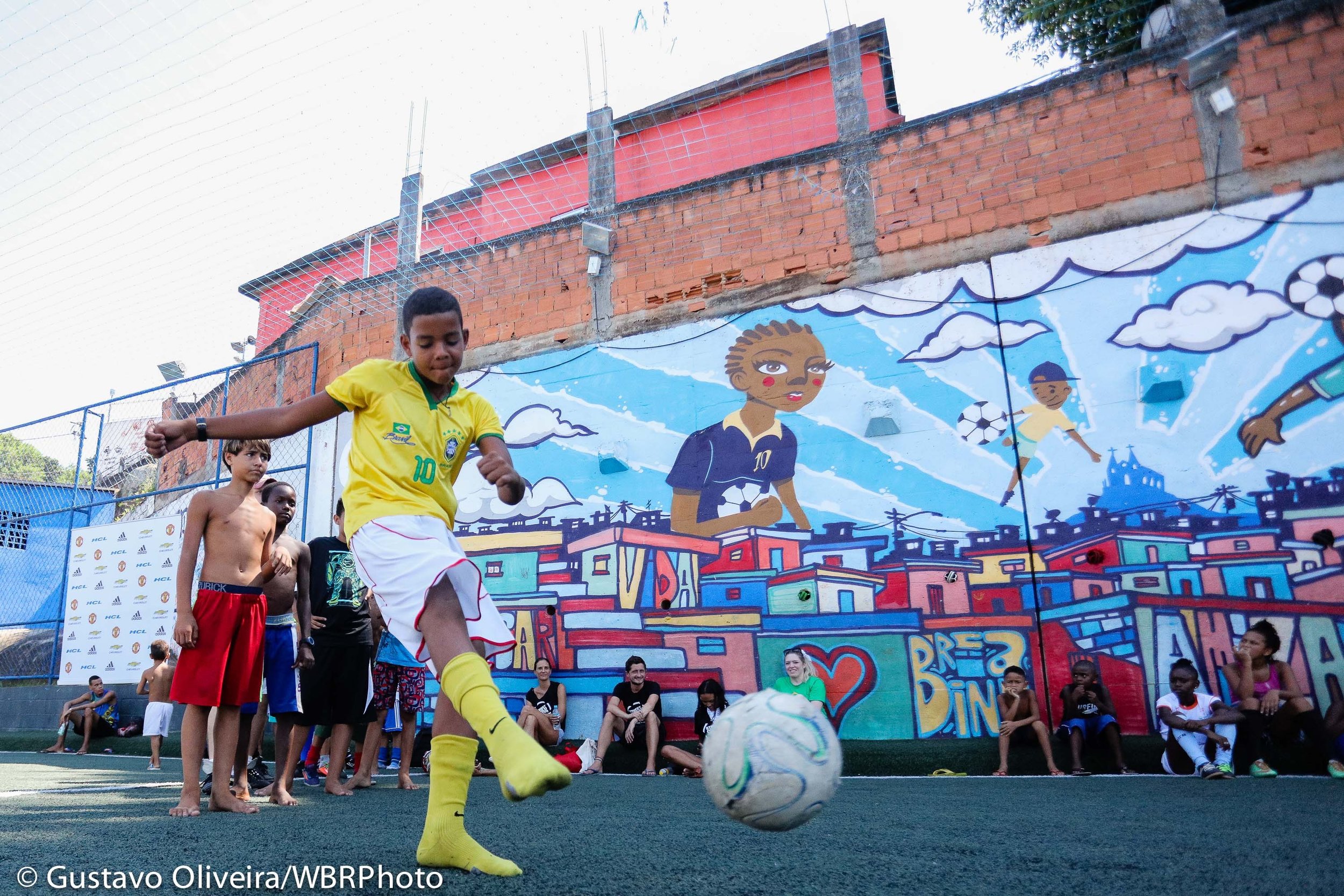In a vibrant public area, a young boy with dark skin and short hair captures the spotlight as he plays soccer, clad in a bright yellow t-shirt, white shorts, and yellow knee-high socks, notably without shoes. The boy is intently focused on kicking a white ball with green stripes, his right foot extended in the air, his body tilted in concentration. Surrounding him are four to five children, visibly watching and possibly waiting their turn to play; two of these children are shirtless, one with red knee-length shorts and the other with blue shorts. The entire scene takes place against a striking mural painted on the side of a building, depicting children of various skin tones playing soccer amidst a backdrop of colorful houses and a cityscape rendered in blues, pinks, purples, reds, whites, and tans. The mural mirrors the live action with an image of a child wearing a yellow shirt and white pants, similar to the central boy. In the background, more children and several adults sit or lean against the mural, seemingly captivated by the game. The sky above is largely unseen, but hints of it suggest a clear, white complexion. The corner of the image bears the copyright of Gustavo Oliveira, WBRP photo.